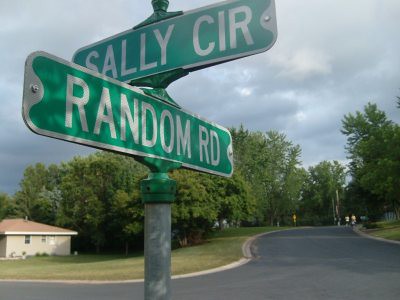This close-up photograph captures an intersection sign in a residential neighborhood. The green street signs with white lettering mark the crossing of Sally Circle and Random Road, affixed to a metal pole. The backdrop features an overcast, gray-blue sky, suggesting imminent rain. Dominating the scene are dense trees lining the intersecting black-topped streets, which lack sidewalks but have concrete gutters. In the lower left-hand corner, a ranch-style tan house with a slightly red-orange tiled roof is partially visible, accompanied by a neatly maintained lawn.